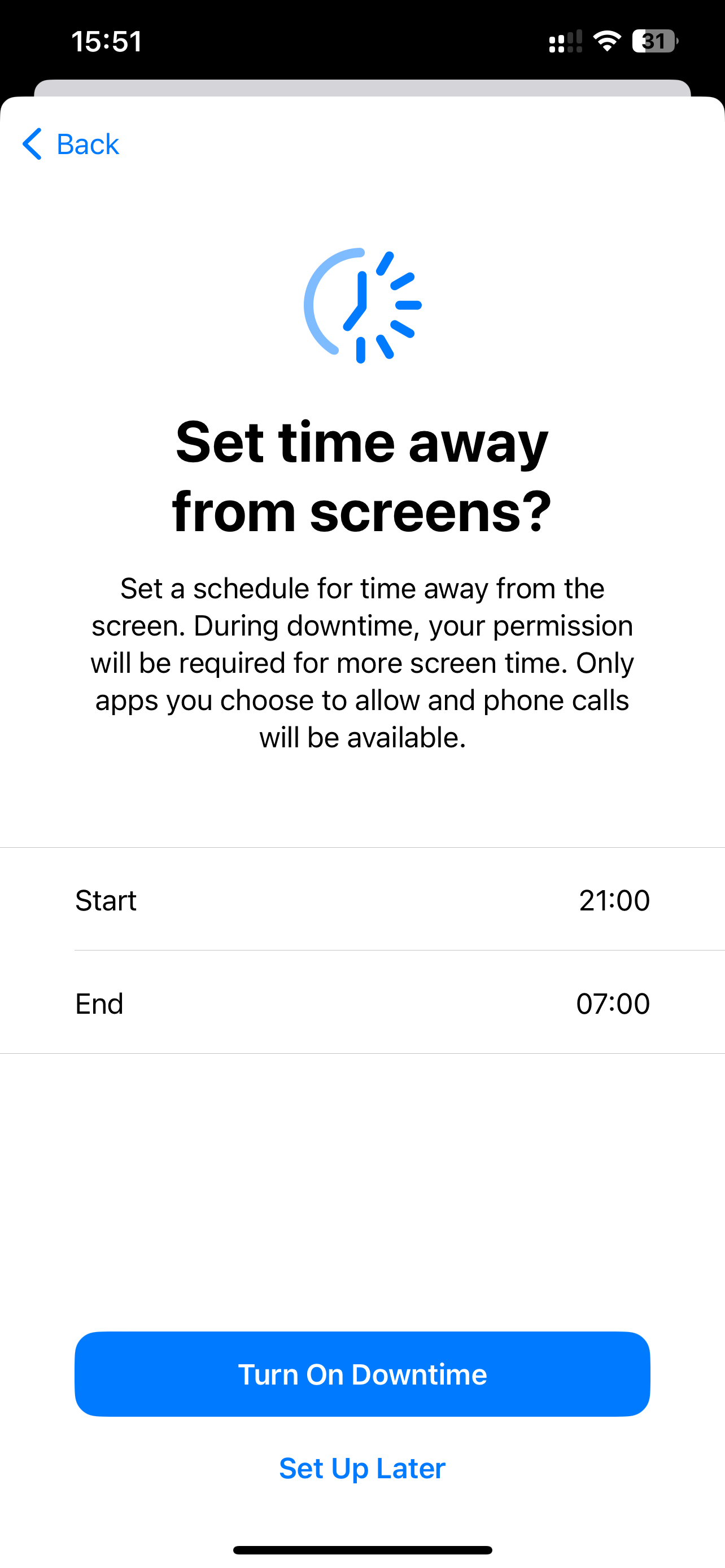The image captures a smartphone screen displaying a settings page for scheduling screen downtime. At the top of the screen, there is a banner showing the current time, "1551," on the left in military format, and the battery life at "31%" on the right.

The page header reads, "Set time away from screens?" followed by detailed instructions in smaller black text: "Set a schedule for time away from the screen. During downtime, your permission will be required for more screen time. Only apps you choose to allow and phone calls will be available." Below, it shows two input fields labeled "Start" set to "21:00" and "End" set to "7:00," indicating the duration for the scheduled downtime.

At the bottom of the screen, a blue rounded rectangle displays the option "Turn on downtime" in white text. Underneath that, still within the white background, there is a smaller blue-text option labeled "Set up later." Additionally, in the top left corner, blue text accompanied by a left-facing arrow provides a "Back" navigation option. The entire page features a clean, white backdrop, highlighting the mentioned elements distinctly.